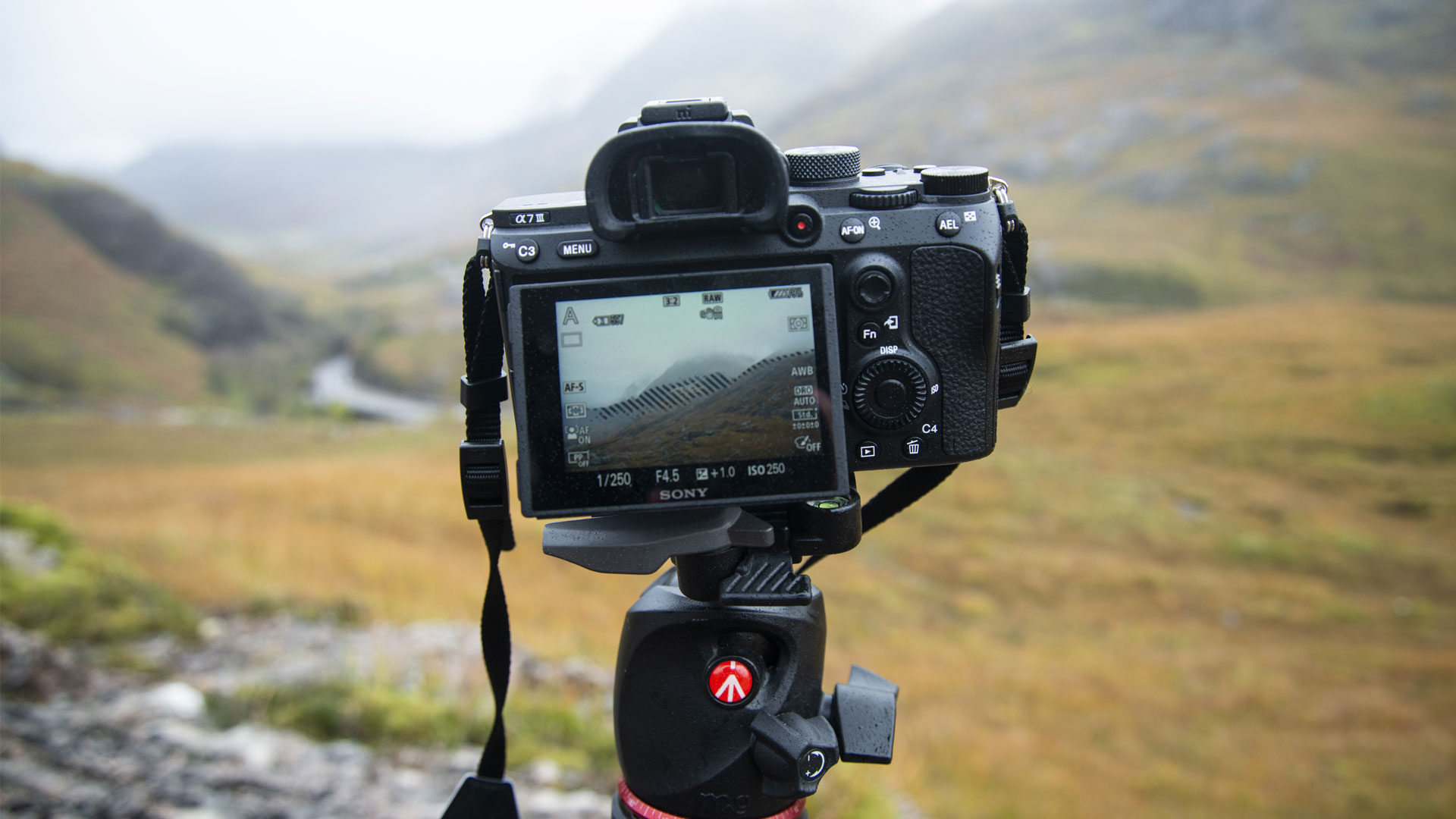This photograph captures a detailed scene of a black Sony DSLR camera set up on a tripod with a white peace sign logo within a red circle. The camera, adorned with various knobs, buttons, and dials labeled "menu" and other settings, is equipped with a neck strap and features a swivel preview window that is currently displaying a landscape view through its lens. The scene it focuses on consists of sprawling valleys, fields, and hills with patches of yellow and green grass, rocks, and a meandering river. The camera’s rear screen is showing white text presets, indicating it is turned on and actively recording. The backdrop is slightly blurred, enhancing the sharpness of the camera itself against the overcast daylight in the mountainous terrain.